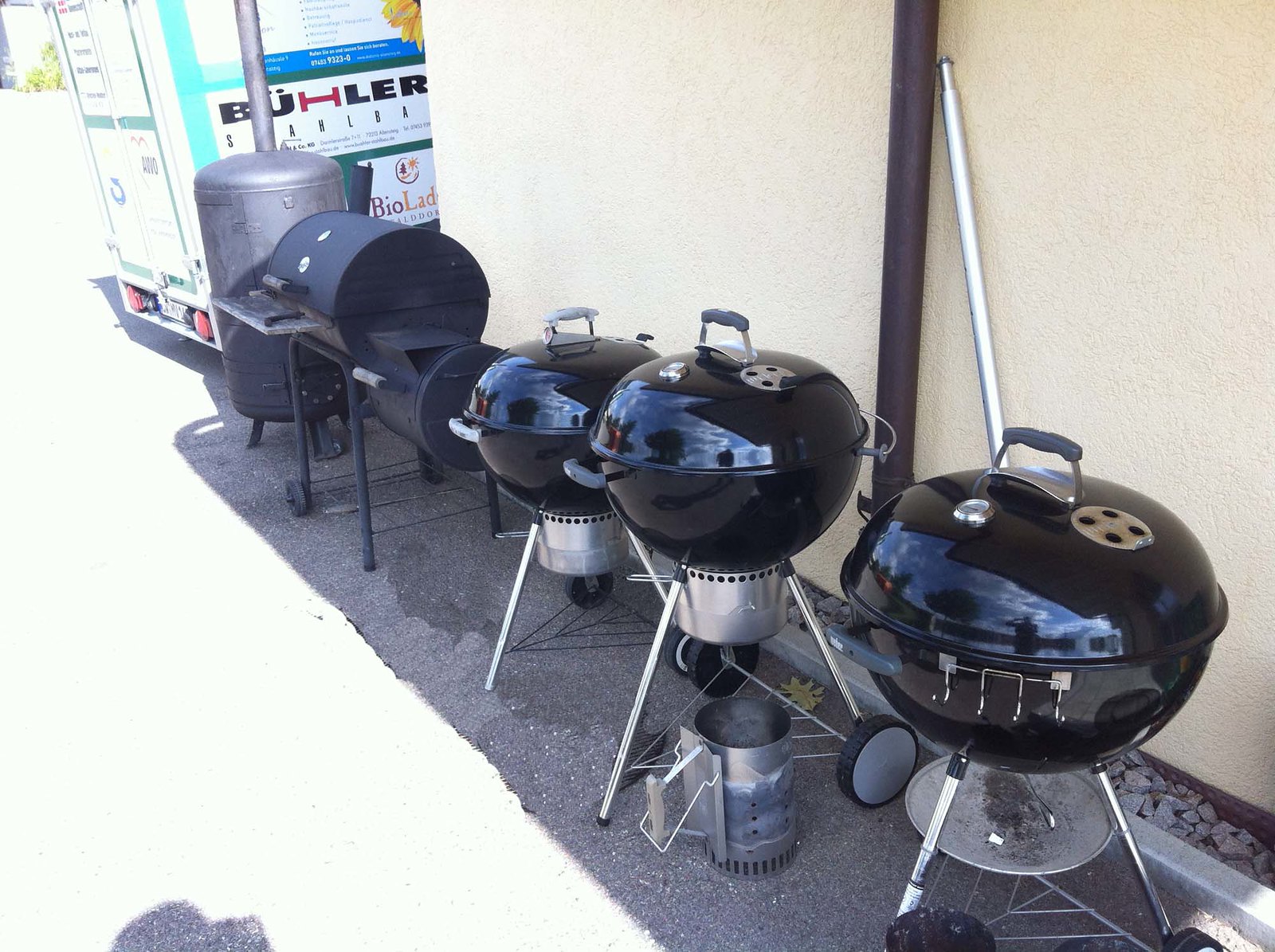In this outdoor photograph, five barbeque grills are lined up against the stucco wall of what appears to be a commercial building, likely a home and garden store. The building features a commercial-grade downspout, indicating its purpose. The grills are situated in the shade, although it's evidently a sunny day outside, as highlighted by the well-lit environment.

To the right side of the lineup, there are three smaller grills, characterized by their simplistic, bowl-shaped, lollipop designs with three prong legs and wheels at the bottom. These grills are fairly standard and could operate on either gas or charcoal. They all share a black color, and one of them has a cylinder space at the bottom, hinting at its multifunctional use. Despite their similar appearance, they vary slightly in size and show minimal signs of use, with the rightmost grill having an ash catcher.

On the left side, there's a large smoker grill with its own smoke unit on the right side, attached to it. This smoker is notably bigger and more complex, featuring a substantial furnace and capable of handling more extensive cooking tasks. An even larger smoker grill stands next to it, distinguished by its imposing size, capable of accommodating significant quantities of food, almost large enough for a person. This too is black in color and adds to the diverse functionality displayed in this array of outdoor cooking equipment.

Adjacent to these grills, the presence of a moving truck parked next to the building accentuates the commercial setting of the scene.